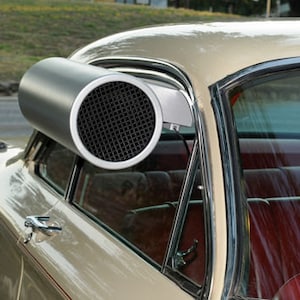This photograph captures a close-up view of a vintage car from the left side, slightly behind the windscreen. The car features a light brown, beige-y paint job that exudes an old-fashioned charm, likely dating back to the 1950s. The car's exterior boasts silver, metal chrome edging around the windscreen and windows, and old metal handles that further enhance its classic aesthetic. The interior reveals dark red leather bench seating that lacks modern seatbelts, suggesting it's a relic from a bygone era. A notable detail is a small triangular window at the front that can be opened with a manual latch.

Affixed to the passenger side window is a somewhat incongruous yet eye-catching silver cylindrical device. This device, which evokes the nostalgic feel of drive-in movie speakers, is mounted parallel to the car's direction of travel. It features a black grill at the front and a boxy extension or chute that secures it to the window. The contraption, which some might mistake for a futuristic speaker or even an aeroplane engine, contrasts sharply with the vintage vehicle it adorns. The background hints at a peaceful setting with a grassy bank barely visible.